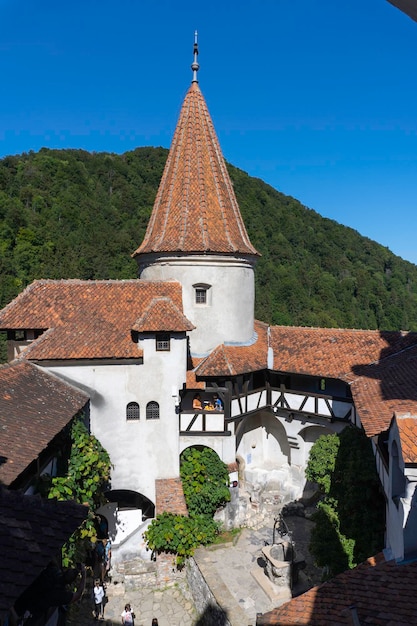The image captures a serene outdoor scene of a small, picturesque village that exudes an old-world charm, possibly situated in an Eastern nation. Dominating the background is a lush, verdant mountain full of trees under a clear blue sky. The village itself features a collection of white and grayish stone buildings with distinctive architectural details, including classic clay-tile roofing. One of the focal points is a striking house with a pointy turret on top, capped with a reddish-orange roof. The house is adorned with small square windows and surrounded by green shrubbery. 

In the village square, which is paved with stone, there is a notable white pillar with a cylindrical shape and an orange and white roof, possibly functioning as a statue or well, with an antenna protruding from its top. The square is also dotted with some green plants. The scene includes three people standing or walking towards the house, seemingly exploring or visiting this timeless place. The rustic ambiance is accentuated by a few missing shingles on the old wood-like roofs, adding to the village's historical and authentic feel.